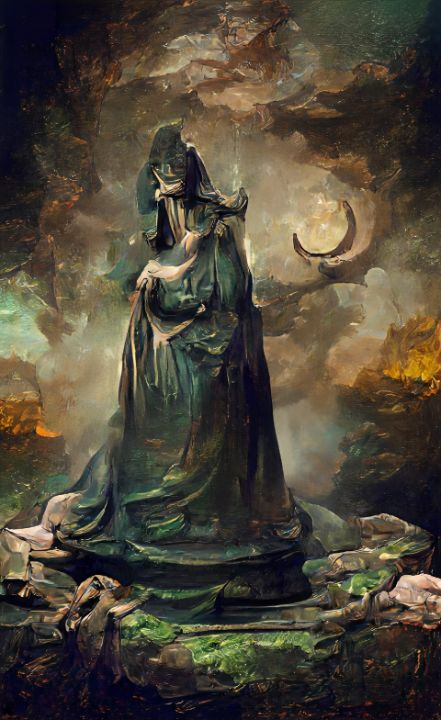The image depicts an abstract, low-resolution painting, resembling an oil painting with a pixelated finish. Central to the piece is a statue-like figure with a nondescript, stone-like face, faintly visible and partially obscured by a headdress or abstract features. The figure, shrouded in a flowing, dark greenish-black robe that features lighter highlights of yellows and beige, appears to rest its hand, which is fashioned from yellow stone, pensively on its chin. The robe billows outwards, widening toward the base, and the figure seems to be positioned on a rocky pedestal surrounded by additional rock formations and greenery. The background encapsulates a swirling array of vivid colors—ranging from oranges, greens, browns, blacks, and yellows—creating a cavernous and cloudy environment. The painterly style of the artwork embraces an abstract, less-defined aesthetic, employing bold colors and fluid shapes to evoke a sense of mysticism and depth.